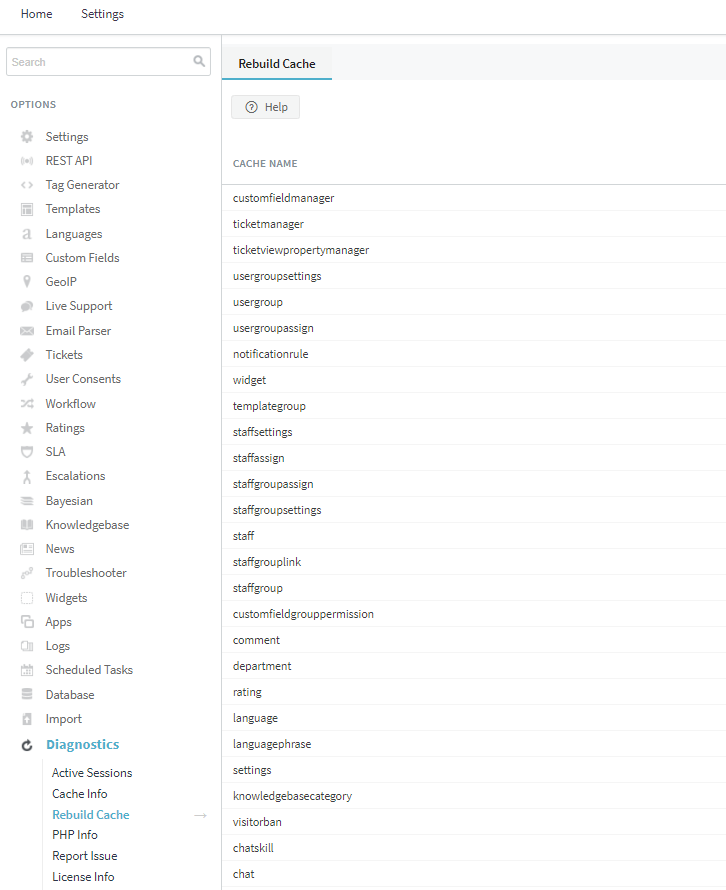An image captures a partial view of a computer screen, roughly covering half to three-quarters of the horizontal span. At the very top of the screen, the words "Home" and "Settings" are visible. Directly below, there's a prominent search bar. Beneath the search bar, a vertical column of multiple lines presents various options. Near the bottom of this column, the word "Diagnostics" appears in blue, followed by a few additional options. Further down, the option "Rebuild Cache" is highlighted in blue.

To the right of this column, the screen shifts focus, displaying the header "Rebuild Cache" at the top. Below this header is a list comprising various titles: "Custom Field Manager," "Ticket Manager," "Template Group," "Department," "Language," "Phrase," and "Settings." In the initial column of options, users see headings such as "Settings," "Tickets," "Email," "Parser," "SLA," and "Escalations." In the "Diagnostics" section, options include "Active Sessions," "Cache Info," and "Report Issue." The "Rebuild Cache" option has been selected, as indicated by its blue highlight.